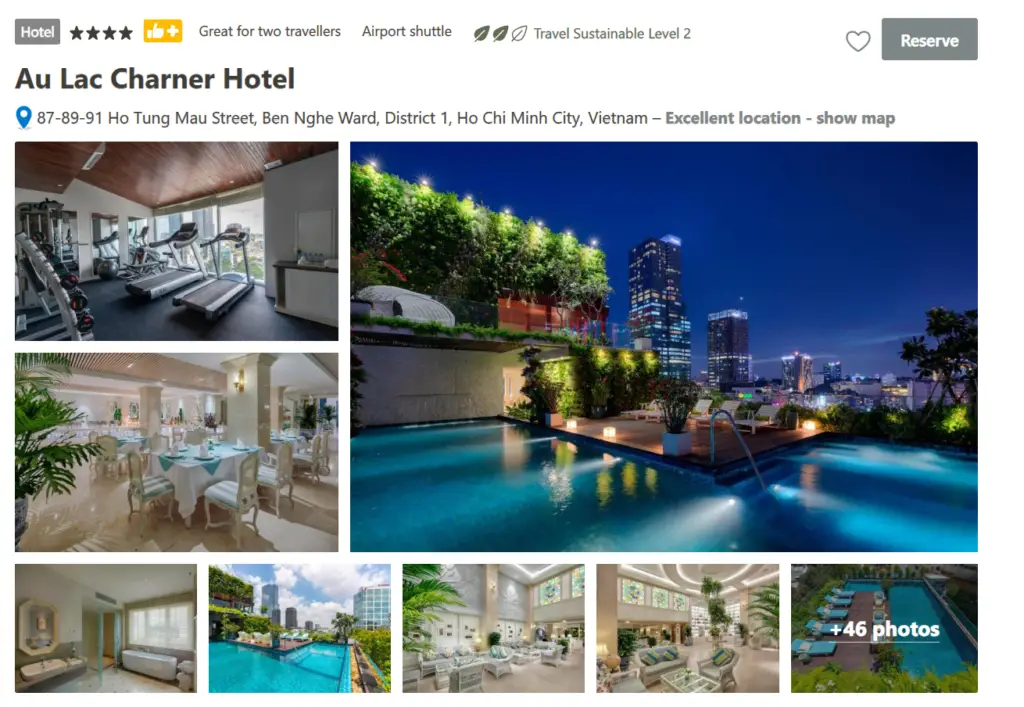The visual advertisement for the A La Charter Hotel prominently features multiple inviting images of the establishment, aimed at highlighting its amenities and exceptional services. 

In the upper left-hand corner, a gray box with white text prominently displays the word "Hotel," alongside a four-star rating. Additionally, there is a thumbs-up symbol with a plus sign, indicating that the hotel is an excellent choice for two travelers. Icons also showcase amenities like an airport shuttle service and a Travel Sustainable Level 2 certification, represented by two black out of three leaves. A heart icon and a gray reserve button are situated to the right.

Returning to the main hotel name on the left, “A La Charter Hotel,” the address is listed as 87-89-91 Ho Tung Mau Street, Binh Ninh Ward, District 1, Ho Chi Minh City, Vietnam, accompanied by a label stating "excellent location" and an invitation to "show map."

In the top-left corner, an image features the hotel's fully equipped gym, showcasing a couple of treadmills and assorted weights. Directly below, another same-sized image depicts a sophisticated dining room adorned with white tables, white tablecloths, and teal accent tablecloths.

To the right, the largest image captures the allure of the outdoor pool, surrounded by lush gardens and offering a picturesque view of the city. At the bottom, a series of five smaller images further detail the hotel’s offerings: the leftmost image shows a room with a mirror and a sink, although partially obscured by a window. The next image provides a daylight view of the pool, further emphasizing the serene atmosphere.

Overall, the ad intricately captures the luxurious and comprehensive nature of A La Charter Hotel, making it a compelling destination for prospective guests.